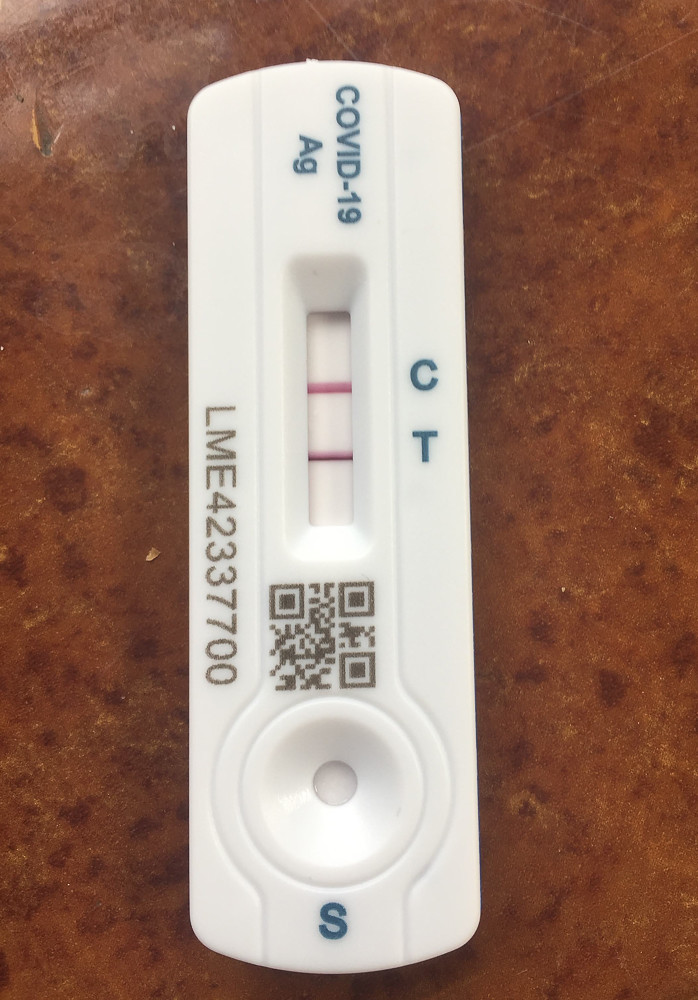A detailed close-up photograph showcases a used COVID-19 test, prominently displaying its white, rectangular form. The test is positioned vertically, enabling the horizontal orientation of the text. At the top of the test, "COVID-19" is clearly printed, followed by "Ag" beneath it. A unique serial number "LME42337700" and a QR code are located along the bottom edge of the device.

Centered in the middle of the test is a port marked with the letter "S," designed for sample insertion. Adjacent to this port is a testing window labeled with the letters "C" and "T" arranged vertically. Both the "C" (Control) and "T" (Test) lines display red markers, indicating that the test has been activated and used.

The test lies on a surface with a reddish-orange-brown stone pattern. Though it is evident the test has been used, it's unclear whether it indicates a positive or negative result. The appearance and arrangement of the lines suggest that a sample has been processed, aligning with observed protocols for such diagnostic tests.